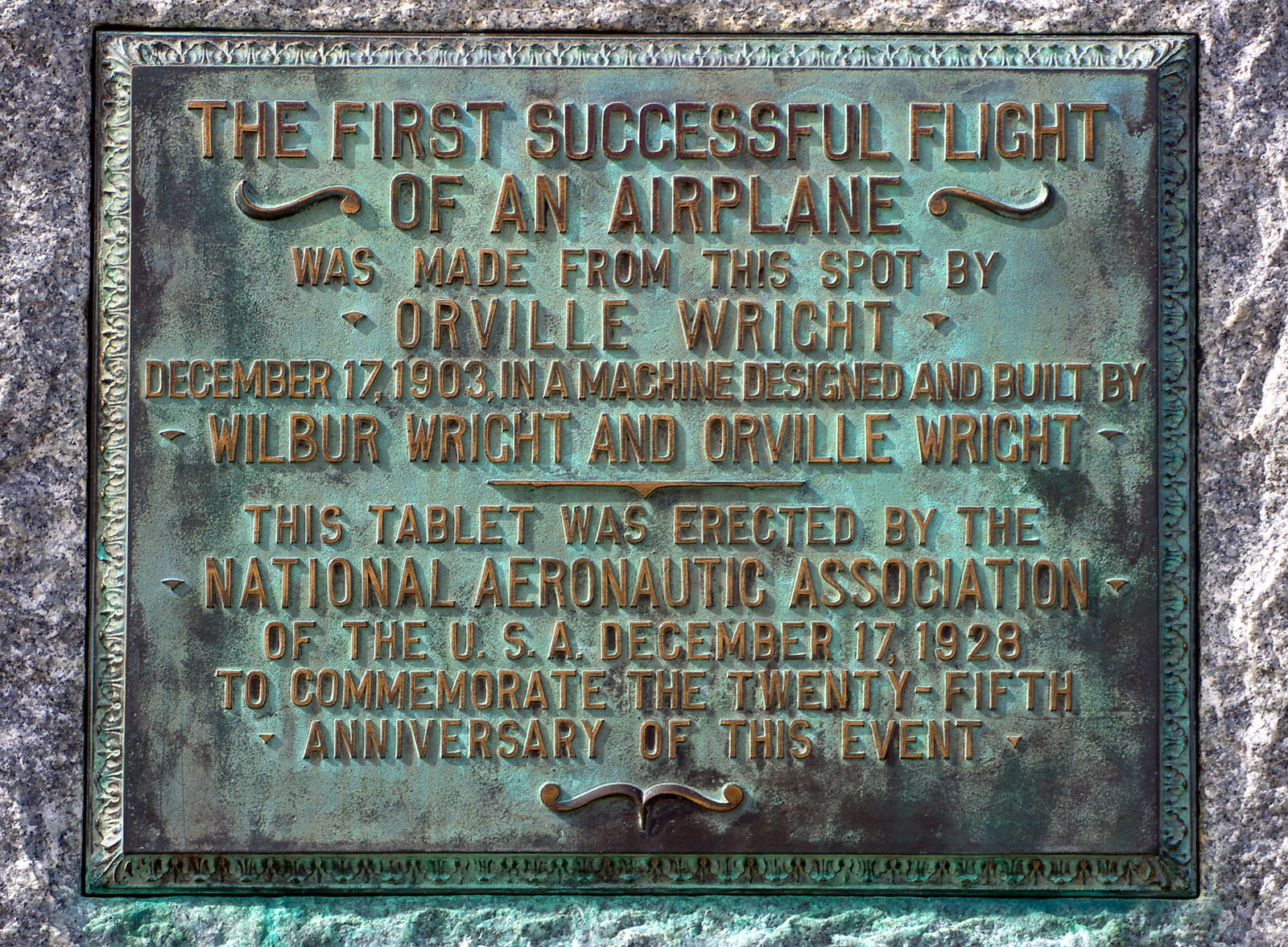This color photograph, taken in landscape orientation, captures a commemorative plaque embedded in a gray granite wall. The bronze plaque, having weathered over time, now displays an aqua-green patina indicative of oxidation, with traces of its original bronze hue still visible, especially around the raised print and ornate fleur-de-lis trim. The stone surrounding the plaque appears in shades of gray, with hints of white and purple colors, particularly at the bottom where the metal has begun to oxidize. The inscription on the plaque reads: "The first successful flight of an airplane was made from this spot by Orville Wright, December 17, 1903, in a machine designed and built by Wilbur Wright and Orville Wright. This tablet was erected by the National Aeronautic Association of the USA December 17, 1928, to commemorate the 25th anniversary of the event." The plaque stands as a testament to a pivotal moment in aviation history, framed by its oxidized elegance against the solid, enduring granite.